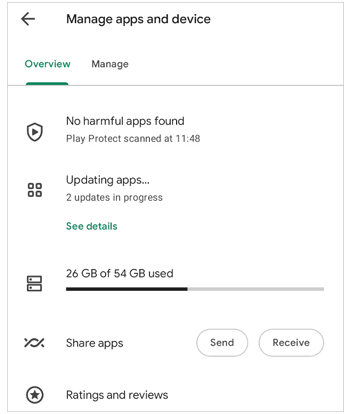This mobile application screen capture, viewed in portrait mode, showcases a minimalist interface primarily set against a white background with black text and icons. The subtle blue-green hue is strategically used to highlight two interactive components: a selected "Overview" tab and a "See Details" button. At the top, a prominent header reads "Manage Apps & Device," below which are two tabs: "Overview" (currently active) and "Manage" (inactive).

The main content area displays five vertically-aligned icons on the left, each accompanied by descriptive text:
1. "No harmful apps found" – reassuring the user of the device's security.
2. "Updating apps" – indicating ongoing updates.
3. "26 GB of 54 GB used" – paired with a black slider bar, visually depicting storage utilization.
4. "Share apps" – featuring "Send" and "Receive" buttons for easy app sharing.
5. "Ratings & reviews" – an invitation to engage with the app community.

The entire screen is framed by a thin gray border, enhancing its clean and straightforward design. The focus on simplicity and essential functionalities suggests an intuitive user experience tailored for efficient app management.